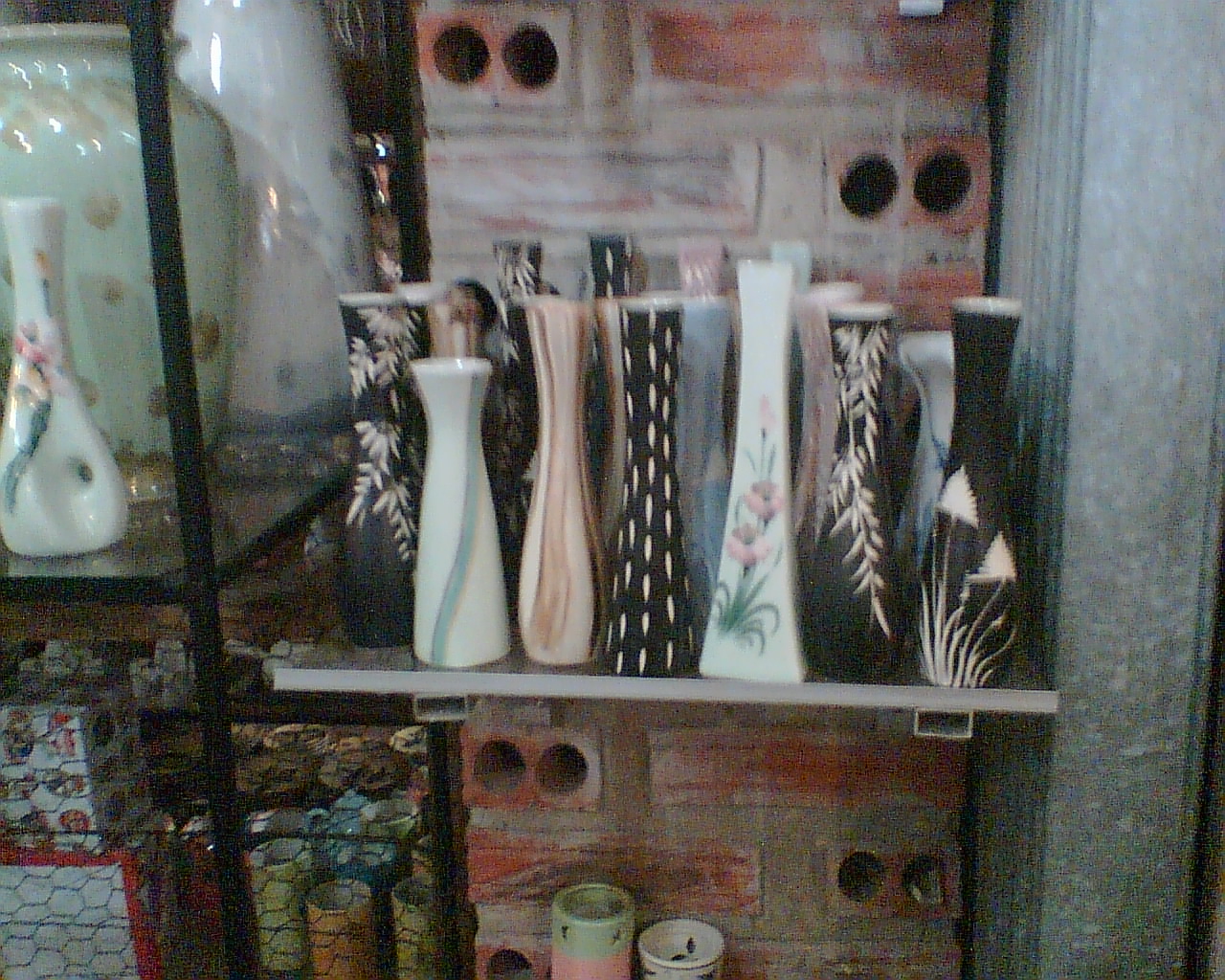This image depicts a collection of narrow, decorative vases displayed on industrial black metal shelving within what appears to be a retail setting, possibly an oriental shop. The shelves are mounted against a red brick wall characterized by bricks with tubular holes drilled through them. The photo itself is blurry and grainy, suggesting low light conditions.

The vases come in various shapes but are all tall and slender, approximately between 6 to 12 inches in height. They feature an assortment of designs; many are black with white leaf patterns, while others include white vases adorned with red and green flowers, and a unique one with a blue diagonal line. Some vases are made from milky swirled glass.

To the left, additional larger vases are displayed on black metal and glass shelves, these vases range from 2 to 3 feet in height. Below the main shelf, a variety of ceramic tea sets and cylindrical glass objects can be seen, likely incense burners or candle holders. The entire setup is densely packed and behind a mesh wire, insinuating it might be the reverse view of an aisle in the store. The shelves to the right are held up by bricks and feature a mix of boxes and more ceramics.